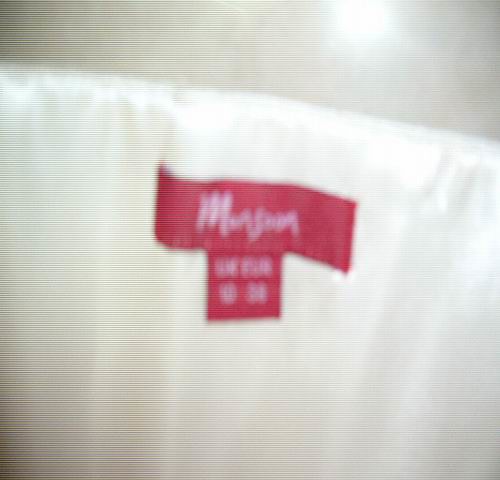This image depicts a very blurry, out-of-focus photograph of a piece of white fabric with a reflective, shiny appearance. The fabric lies against a tan-colored background, which could be a floor tile or wall reflecting a bright light, making the fabric appear extra bright. The focus of the image is a red, rectangular clothing tag sewn onto the fabric. The tag, which looks wrinkled and slightly bent, features white text in a cursive font beginning with an 'M,' likely reading 'Monsoon.' Beneath this main tag, there is a smaller square tag listing sizing information, with 'UK 10,' 'Euro 34,' and possibly additional sizing details, although the text is quite illegible due to the blurriness. The corners of the image appear darker, with shades of black.